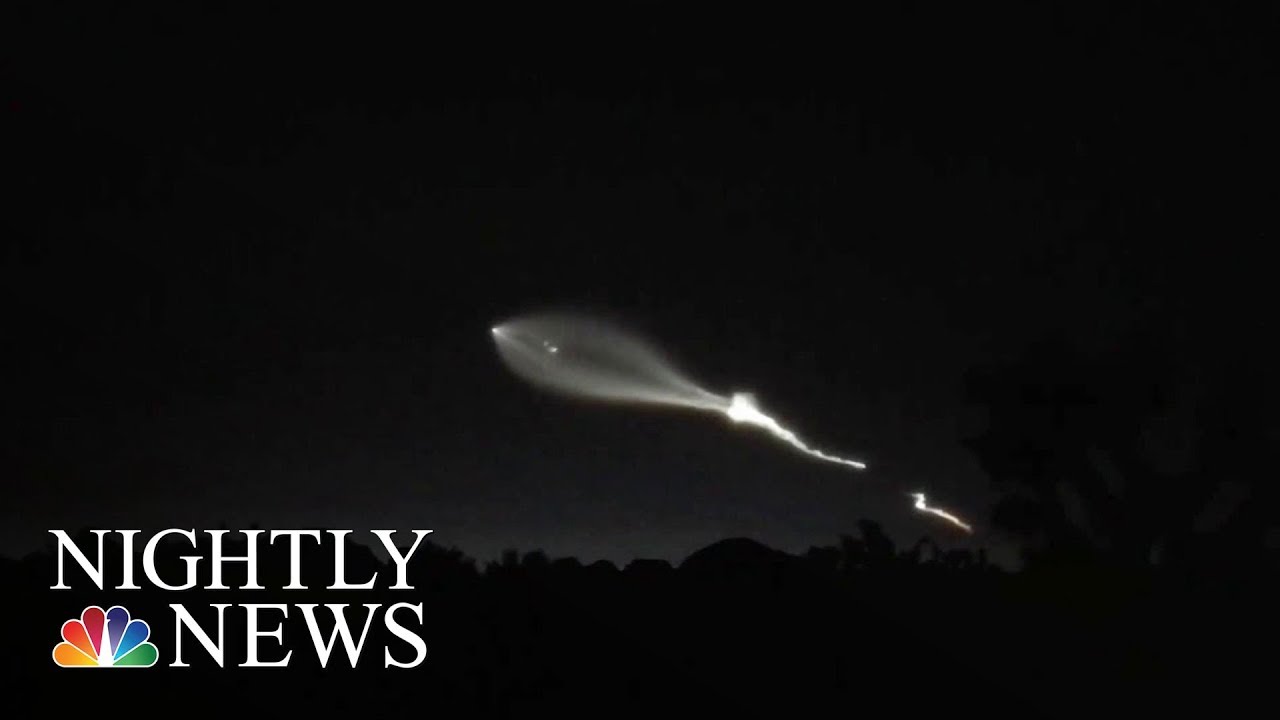The image depicts a dark night sky with a predominant black backdrop. In the center, a bright white streak of light travels upwards to the left, starting larger on the left and tapering off as it moves right, growing brighter towards the tip. The light source has a fragmented yet continuous trail, suggesting the motion of a meteor, comet, or possibly a rocket. The exact nature of the object remains ambiguous, but it exudes a sense of sci-fi wonder, almost akin to a UFO. Silhouettes of trees are faintly visible against the gray-black gradient of the sky, alongside a tiny, mysterious red dot resembling a star. At the bottom left, in white text, "Nightly News" is prominently displayed next to the colorful peacock logo of CNBC, marking the image as a screen capture from the NBC Nightly News broadcast.